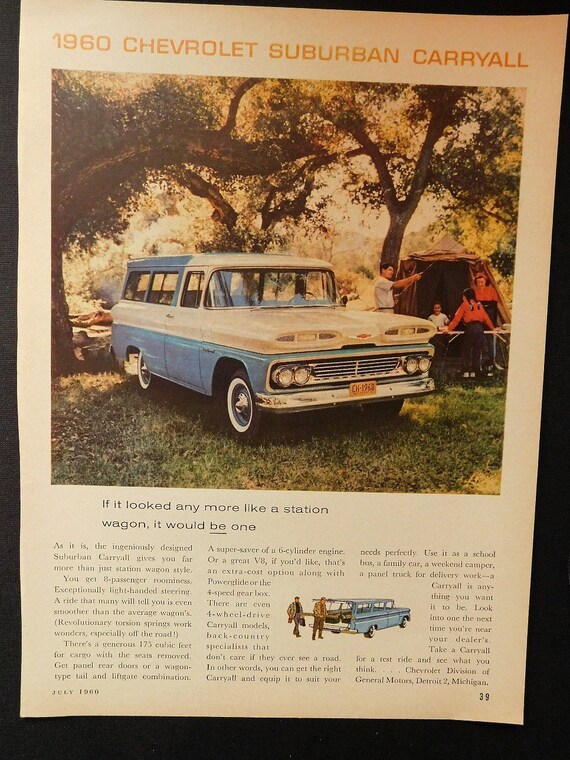This is a detailed photograph of an advertisement page seemingly torn from a vintage magazine dated July 1966, with the page number 28 or 39 visible in the corners. The magazine page has a yellowed tint, suggesting its age. At the top, bold orange text announces the "1960 Chevrolet Suburban Carryall". The ad features a blue and white Chevrolet Suburban with whitewall tires, parked at a campsite amidst spreading oak trees with green and slightly yellowing leaves, forming a canopy over the car. The campsite scene includes a family of four: a father in a t-shirt and beige pants appears to be setting up a tent or rod, while the mother and two children, wearing red and white shirts with dark-colored pants, are gathered around a picnic table near a brown tent. One child is under the tent. The license plate on the Suburban reads "CH 1968", and beneath the image, a caption humorously notes, "If it looked any more like a station wagon it would be one," hinting at the early evolution of the SUV.